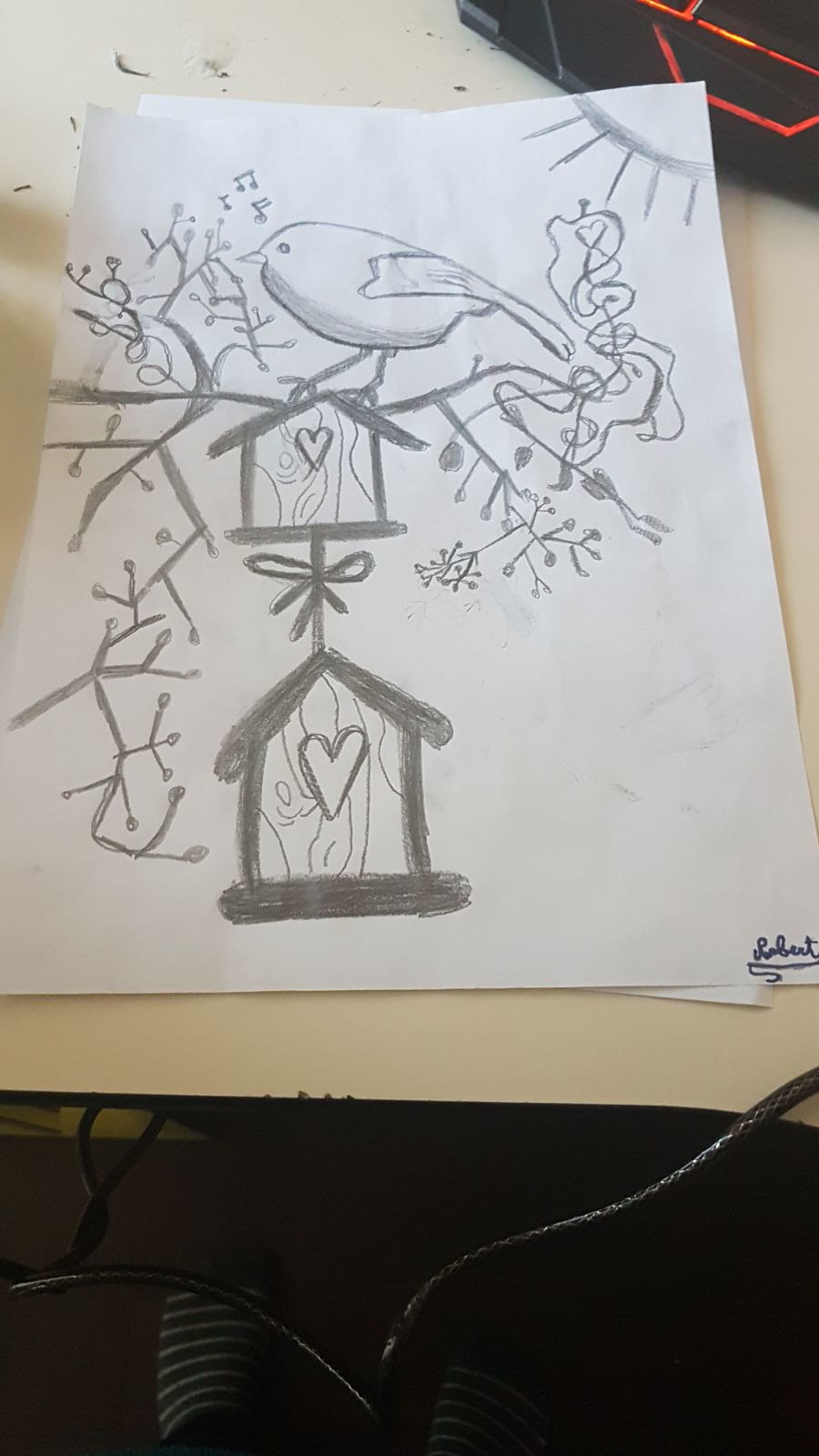The image showcases a meticulously hand-drawn, black-and-white sketch resting on a table. The drawing features an array of detailed elements, starting with a collection of trees emerging from the left side of the paper. These trees appear intricately sketched, demonstrating the artist's attention to natural details. In the upper right corner, about a quarter of a radiant sun is penciled in, casting an implied light over the scene. 

Prominently placed within the foliage is a birdhouse, adorned with a heart at its center. Just below it, a slightly larger birdhouse is similarly decorated with another heart. Atop this birdhouse rests a large bird, one wing outstretched as if in motion. From the bird's beak, a series of musical notes ascend, suggesting a melodious song being sung. The artist's signature at the bottom completes the piece, adding a personalized touch. The entire drawing sits on a flat table surface, providing a backdrop that emphasizes the artwork's intricate lines and thoughtful composition.